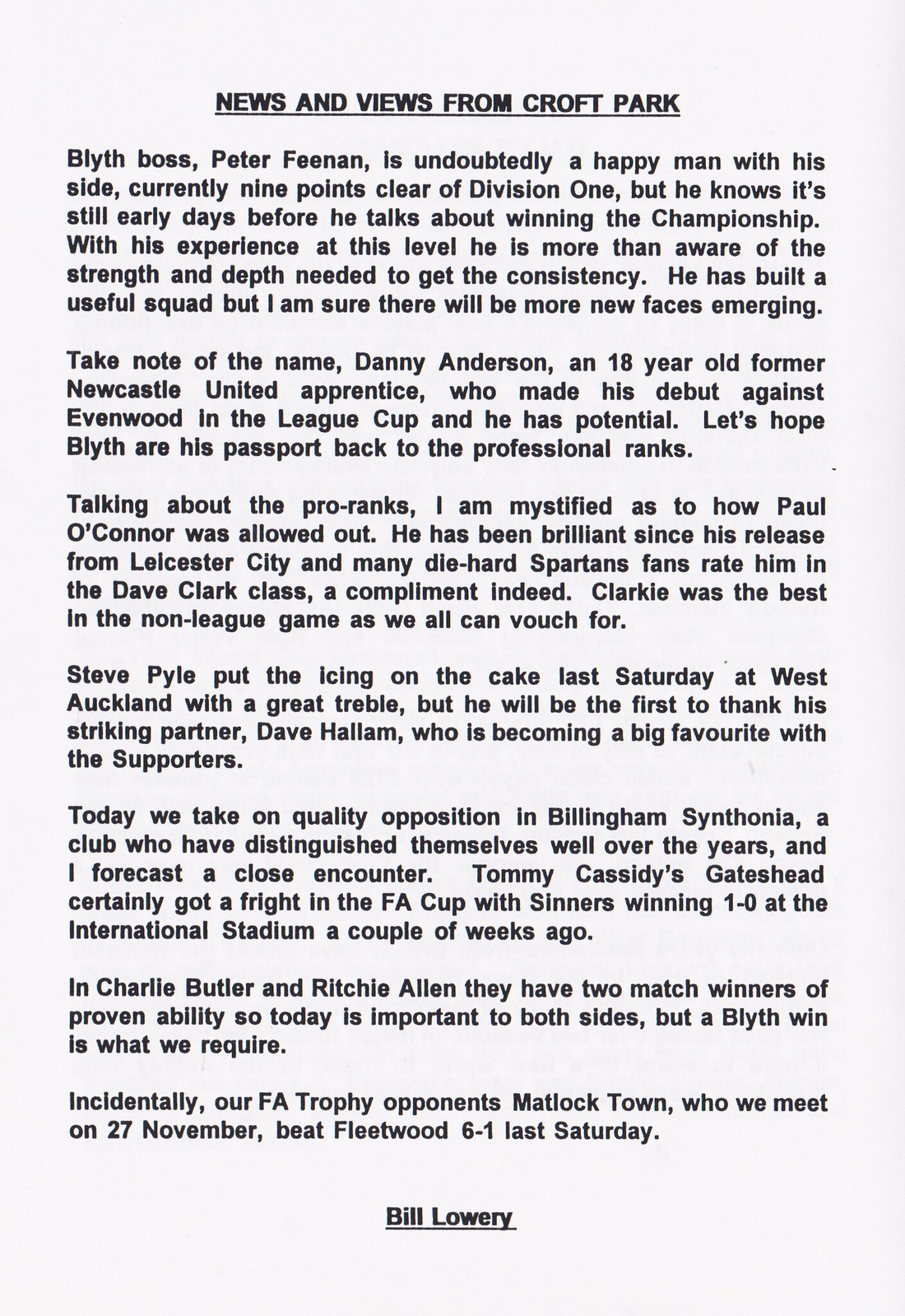The image shows a detailed and comprehensive article titled "NEWS AND VIEWS FROM CROFT PARK," authored by Bill Lowery. The article, printed in black type on a white background, spans seven paragraphs and covers the current state of the Blyth Spartans football team. It starts by highlighting that Blyth's boss, Peter Freeman, is pleased with his team, which is nine points clear at the top of Division 1. Despite the promising lead, Freeman remains cautious about prematurely discussing their championship prospects, emphasizing the need for strength and depth to maintain consistency. 

The article also introduces several key players, including Danny Anderson, a promising 18-year-old former Newcastle United apprentice who made his debut against Evenwood in the League Cup, and Paul O'Connor, who has been outstanding since his release from Leicester City. The author notes how O'Connor is highly regarded by the fans, comparing him to the legendary Dave Clark. Furthermore, Steve Pyle's recent hat-trick at West Auckland is celebrated, with a nod to his striking partner Dave Halam, who is becoming a fan favorite.

As the article progresses, it previews an upcoming challenging match against Billingham Synthonia, predicting a closely fought contest. The author also references a notable past victory by Synthonia against Tommy Cassidy's Gateshead and highlights the proven talent of Charlie Butler and Richie Allen. Finally, the article mentions an upcoming FA Trophy match against Matlock Town, who recently defeated Fleetwood 6-1. The article concludes with the underlined byline of Bill Lowery.